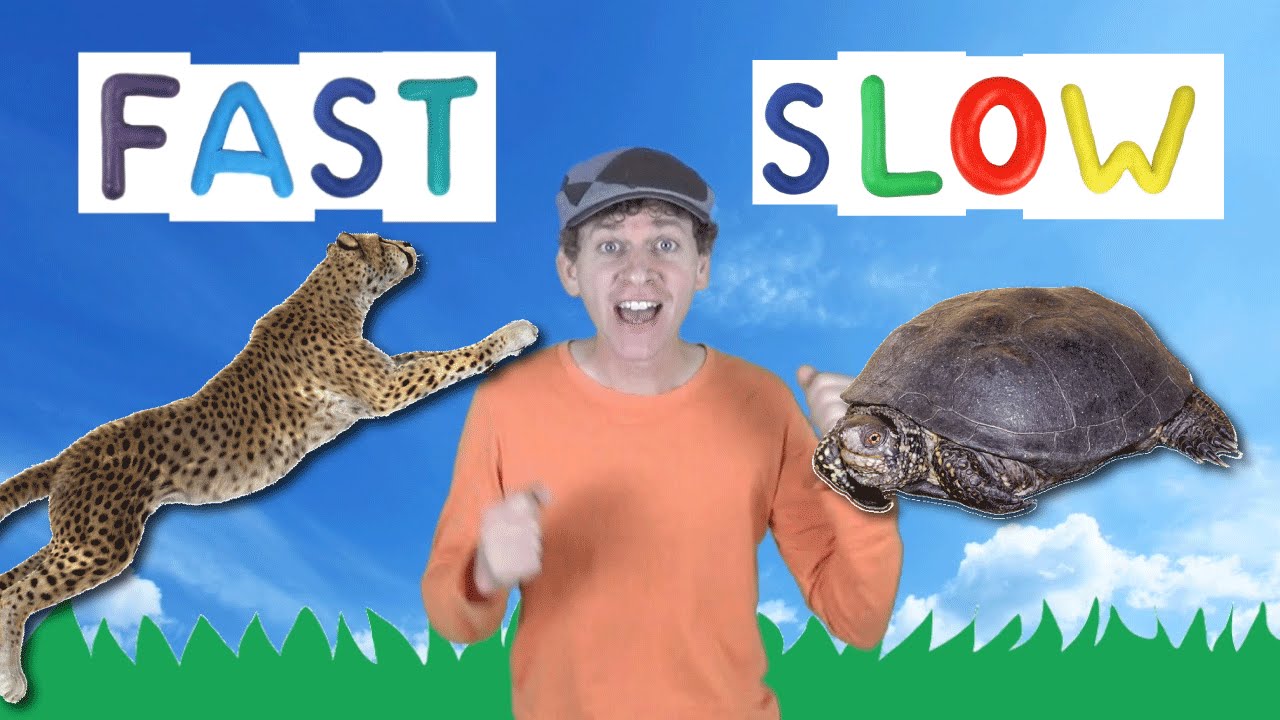The image is a screen capture from a children's YouTube video, likely a thumbnail. It features an enthusiastic white man with a grayish-blue cap and a light orange long-sleeve t-shirt, standing slightly off-center. His mouth is wide open in a smile, suggesting he's excited. The background is a blend of a real photo of a bright blue sky and cartoon grass at the bottom. In the foreground, there is a cutout of a cheetah beneath a sign that says "FAST" on the top left, and a turtle beneath a sign that says "SLOW" on the top right. Each letter of the words "FAST" and "SLOW" is capitalized and in a different color: "FAST" uses purple, light blue, navy blue, and teal, while "SLOW" is depicted in navy blue, green, red, and yellow. The man appears to be illustrating the concept of speed to children, using the cheetah and turtle, animals traditionally known for being fast and slow, respectively.